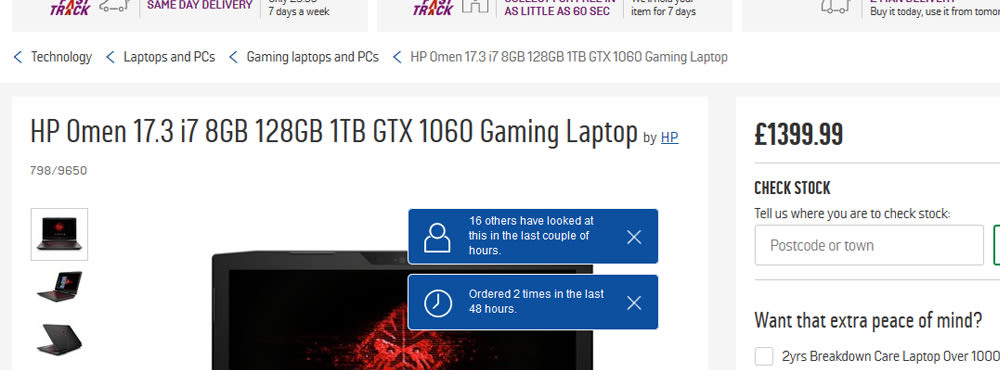In this image, we see a partially displayed webpage that appears to be an online retail platform for technology products. The primary focus is on the "HP Omen 17.3" Gaming Laptop, featuring a 17.3-inch screen, an Intel i7 processor, 8GB of RAM, a 128GB SSD, a 1TB HDD, and a GTX 1060 GPU. The price listed for this high-performance gaming laptop is €1,399.99.

At the top of the page, navigation options are visible, including categories such as “Laptops and PCs” and “Gaming Laptops and PCs,” leading to the featured HP Omen 17. To the right of the product description, the price is prominently displayed.

On the left side of the page, there are three smaller thumbnail images of the laptop, and a larger, but partially cut-off, image showcasing the device. Blue notification pop-ups indicate the product's popularity, with messages such as “16 others have looked at this in the last couple of hours” and “ordered two times in the last 48 hours.”

Furthermore, there is a section for checking stock availability and an area offering extended warranty options, touting “two years of breakdown care for laptops over $1,000.” The webpage features a clean layout dominated by white and grey tones. The text is in black, making it easy to navigate and read through the product details and additional offers.